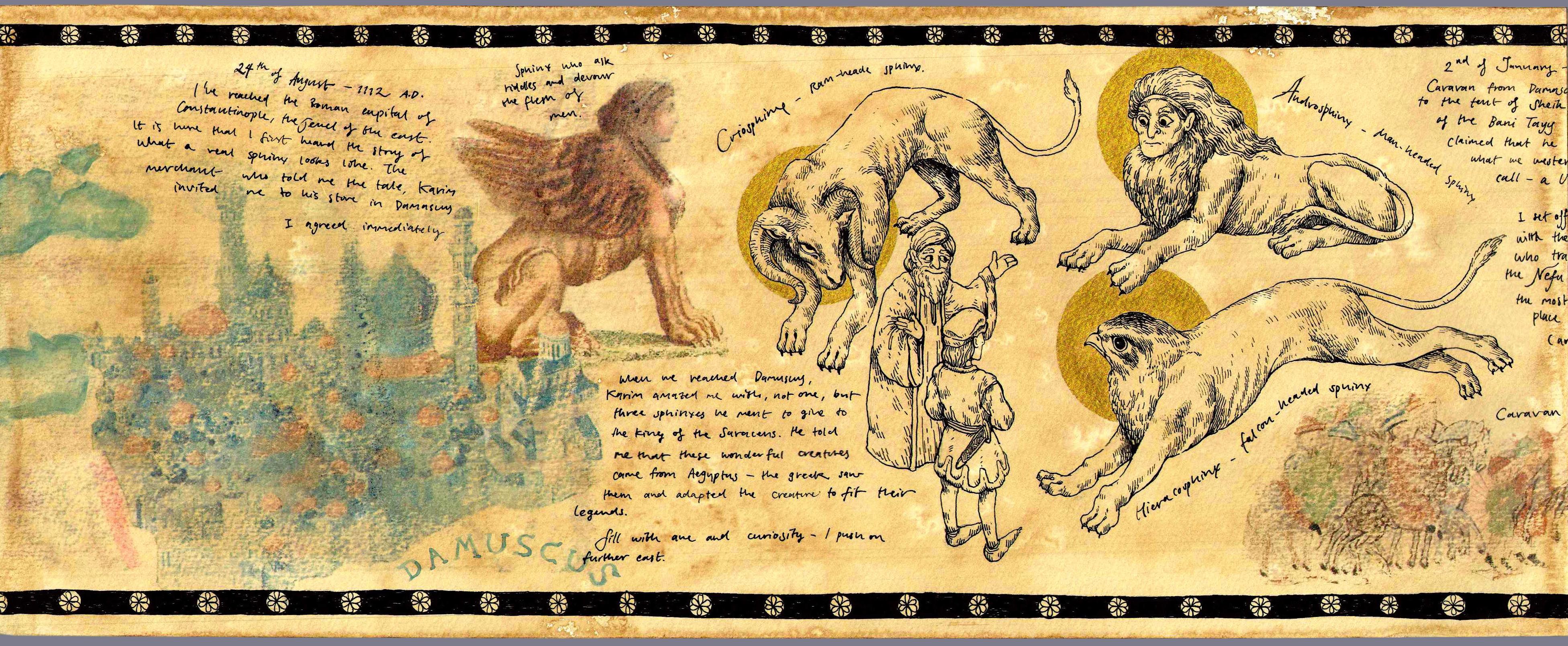This image depicts a weather-worn, triangular-shaped banner or scroll bordered in black with white floral spots. The central artwork features various mythological hybrid creatures with lion bodies that are combined with different heads: a sheep, a bird, a ram, and a human. Some of these creatures also have wings. Interwoven with these fantastical beings are faint gold and light blue hues, adding to the aged, mystical aura of the piece. There is also black ink writing that appears to describe the creatures shown. The entire layout conveys an intricate scene reminiscent of ancient, mythical artistry. Specific details include a reoccurring theme of lions with human and bird heads, a border with black and circular elements, and an overall appearance of old, rusted paper.